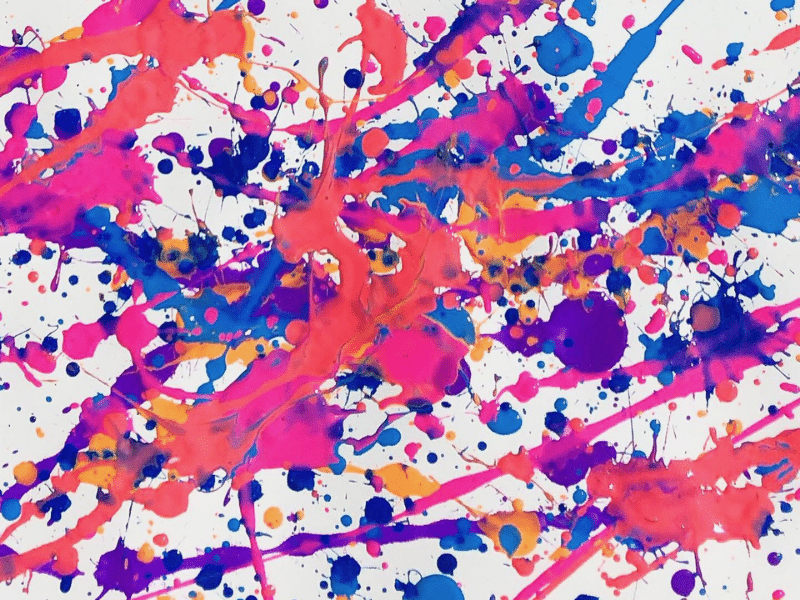This artwork features a white square canvas, prominently displaying an array of vibrant colors created through splatters, streaks, dots, and splotches of paint. Dominated by shades of red, pink, blue (both light and dark), orange, and multiple hues of purple, the piece is an exemplar of abstract or modern art. The random placement of paint suggests an energetic and carefree application, as though the artist repeatedly flicked paint from their hands or brushes, without any discernible brush strokes. Despite its seemingly chaotic creation process, the piece is well lit and captures the essence of spontaneous expression. Whether perceived as a profound artistic statement or a burst of unrestrained creativity, it exemplifies a genre that fascinates many, often commanding substantial monetary value in the art world.